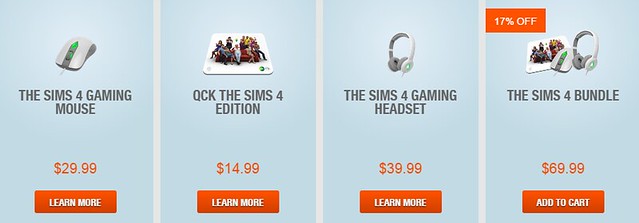This image is a screenshot from the popular game, The Sims 4, showcasing a set of four promotional products arranged in separate rectangular sections. Each section highlights a specific piece of gaming hardware or bundle offer:

1. The first rectangle features "The Sims 4 Gaming Mouse". The mouse is light gray and dark gray with a green light. It's priced at $29.99, displayed in a red rectangle. Below the price, there is a small, white rectangular button labeled "Learn More".

2. The second rectangle displays "QCK: The Sims 4 Edition". The image shows what appears to be game-themed artwork with numerous Sims characters. It is priced at $14.99, also shown within a red rectangle, accompanied by a similarly formatted "Learn More" button.

3. The third rectangle presents "The Sims 4 Gaming Headset". The headset is depicted in shades of gray. The price is $39.99, marked in a red rectangle with the "Learn More" button beneath it in white text.

4. The fourth rectangle advertises "The Sims 4 Bundle". At the top, a small rectangle indicates a 17% discount in white text. This bundle includes all three previously mentioned items: the gaming mouse, the gaming pad, and the headset. The bundle is priced at $69.99 in red text. Below the price, there’s a red "Add to Cart" button with white lettering.

Overall, the image promotes a special sale on these exclusive, game-themed accessories, emphasizing the discounted bundle offer.